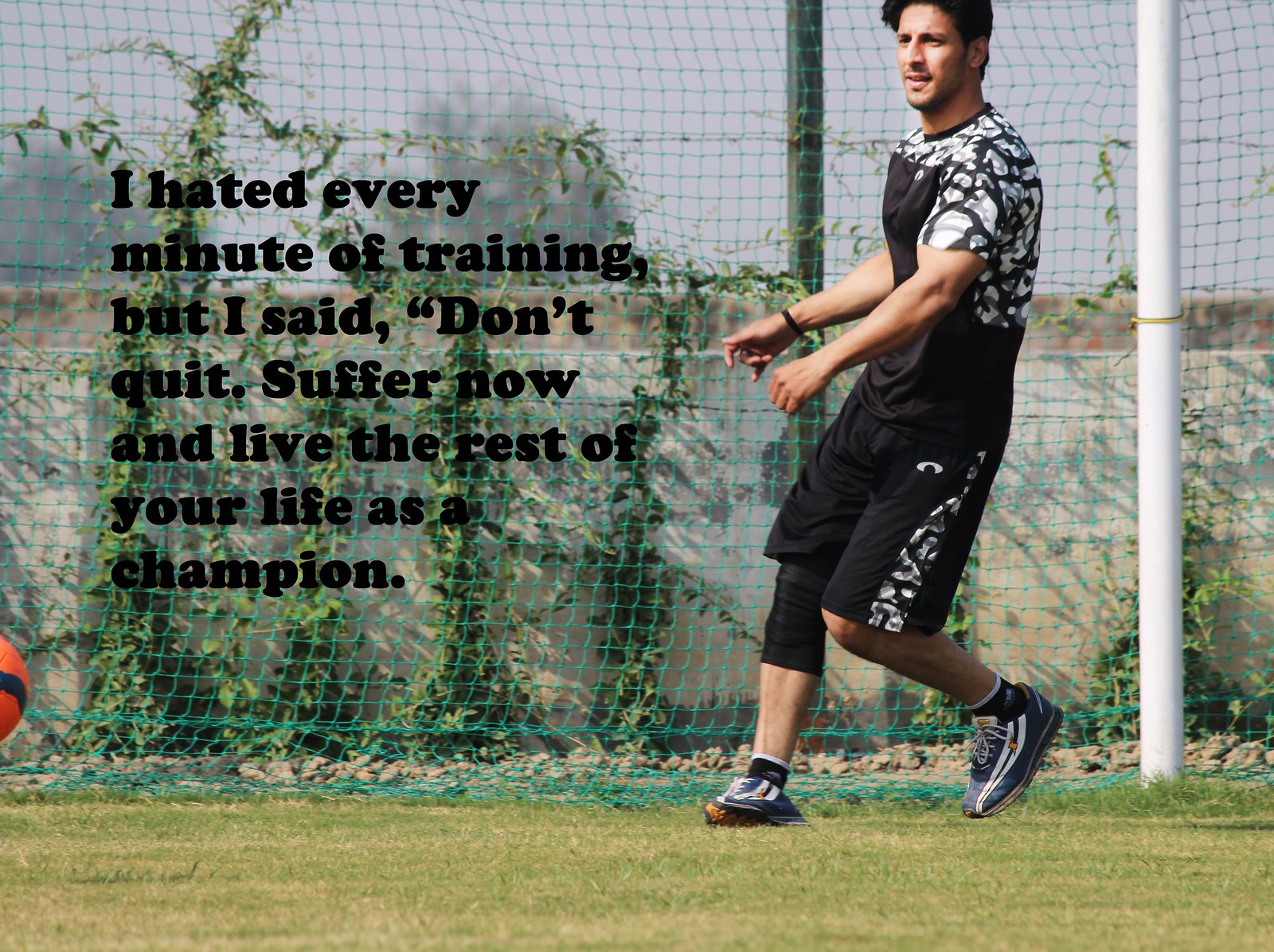In this color photograph, the landscape-oriented image features a young, handsome, muscular man standing slightly to the right of center, in a dynamic pose with his arms outstretched and looking towards the left. He has dark hair and is dressed in a black t-shirt with white prints, black long shorts, black sports shoes, a black kneecap on his right knee, and a black bracelet on his right wrist. The setting is a grassy football field on a sunny day, with a bright blue sky overhead. 

Behind him, a green net with white and green vertical goal posts frames the image, and to the left, partially visible in the corner, is an orange (likely red) soccer ball. Further in the background, plants and bushes add greenery to the scene. Overlaying the bottom left portion of the net is bold black text that reads, "I hated every minute of training, but I said, 'Don't quit. Suffer now and live the rest of your life as a champion.'" This blend of representational realism and graphic typography gives the image a motivational atmosphere.